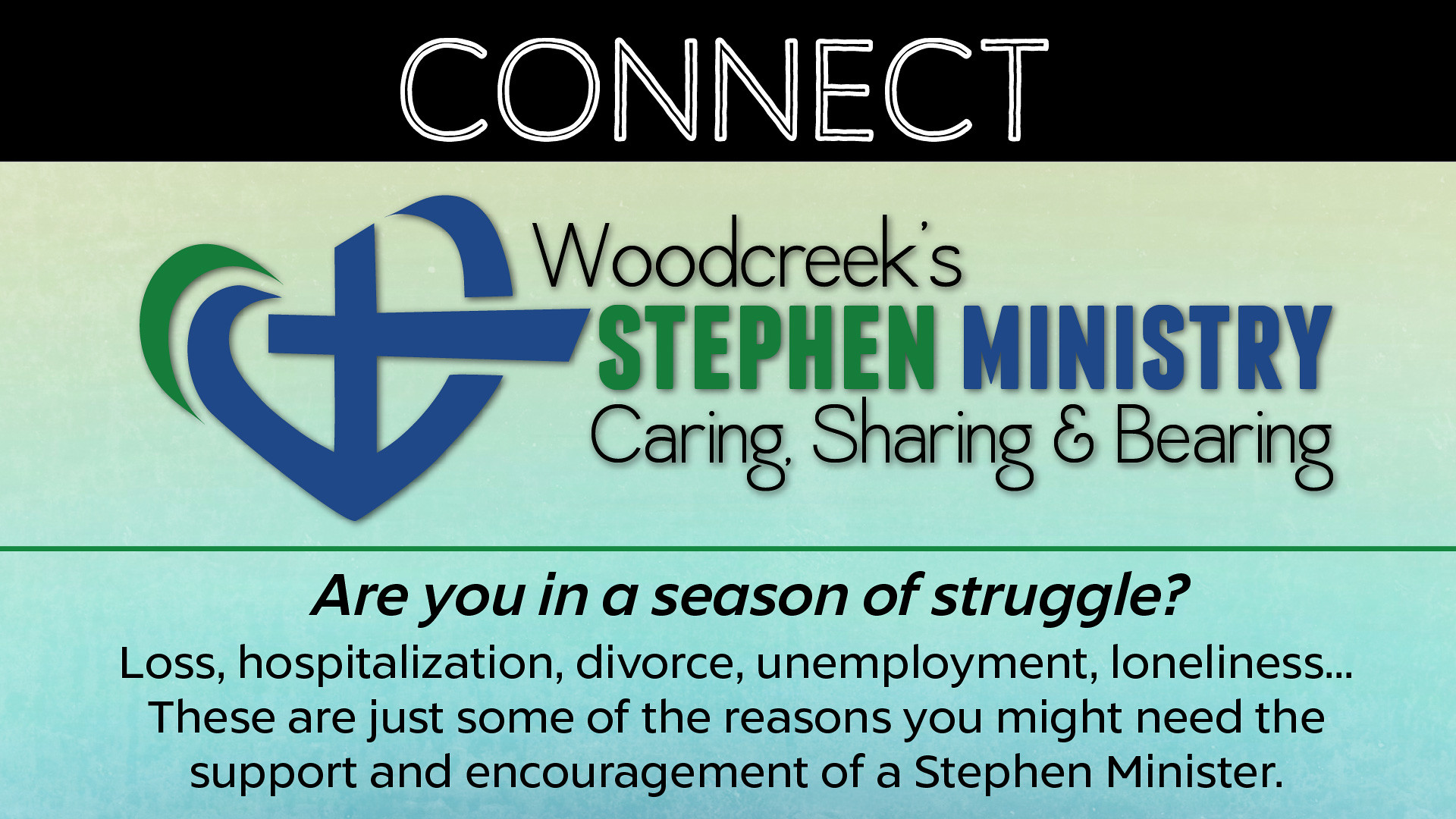The image is a digitally crafted informational poster primarily dominated by text and serving as an advertisement for a church's support services. At the top, a black banner extends across the screen with the word "CONNECT" centered in bold white letters. Below this, the background transitions to a light bluish-green hue. Positioned centrally is a large, distinct blue and green logo featuring a cross. To the right of the logo, the text "Woodcreek's Stephen Ministry" is presented with "Woodcreek's" in green, "Stephen" in blue, and "Ministry" in black letters. Directly under this title, a motto reads "Caring, Sharing, and Bearing" in black text.

The bottom section of the poster addresses potential viewers directly with a probing question in bold black writing: "Are you in a season of struggle?" This is immediately followed by a list of challenges— "Loss, Hospitalization, Divorce, Unemployment, Loneliness..."—presented in a slightly smaller black font. The message continues, explaining that these are just a few reasons why someone might need the "Support and Encouragement of a Stephen Minister." The poster's overall design ensures that the content is well-spaced, offering a clear and accessible call to action. The color palette includes black, white, yellow, blue, green, and gray, creating a balanced and inviting look.